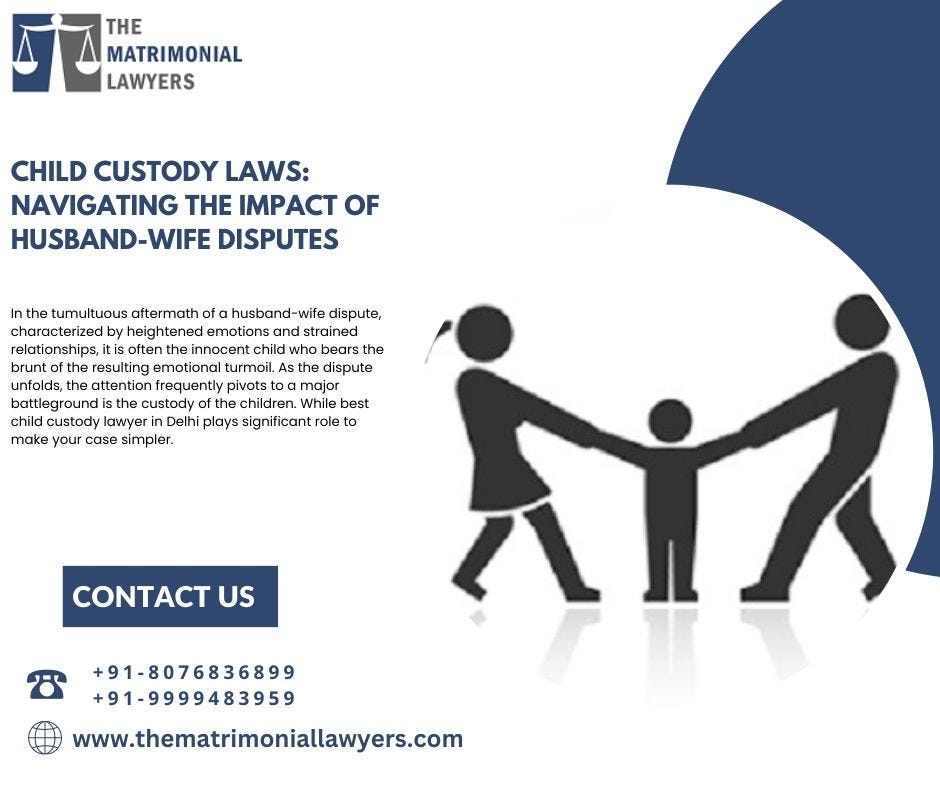The image is a detailed advertisement for matrimonial lawyers specializing in child custody disputes. It prominently features a logo in the top left corner, depicting the Scales of Justice on a blue and gray background, with the text "The Matrimonial Lawyers" next to it. Below the logo is a headline that reads, "Child Custody Laws: Navigating the Impact of Husband-Wife Disputes," followed by a substantial narrative discussing the emotional toll on children and the complexities of custody battles. The primary visual on the right side of the image shows three stick figures: a smaller one in the center representing a child, with a female and a male stick figure tugging at each of the child's arms, emphasizing the conflict. The overall color scheme includes a predominantly white background with black text, complemented by navy blue elements. At the bottom left, there is a blue "Contact Us" button accompanied by a telephone icon, two phone numbers, and the website URL "TheMatrimonialLawyers.com," all highlighted in navy blue. The illustration underscores the emotional and legal struggles involved in child custody cases amid parental disputes.